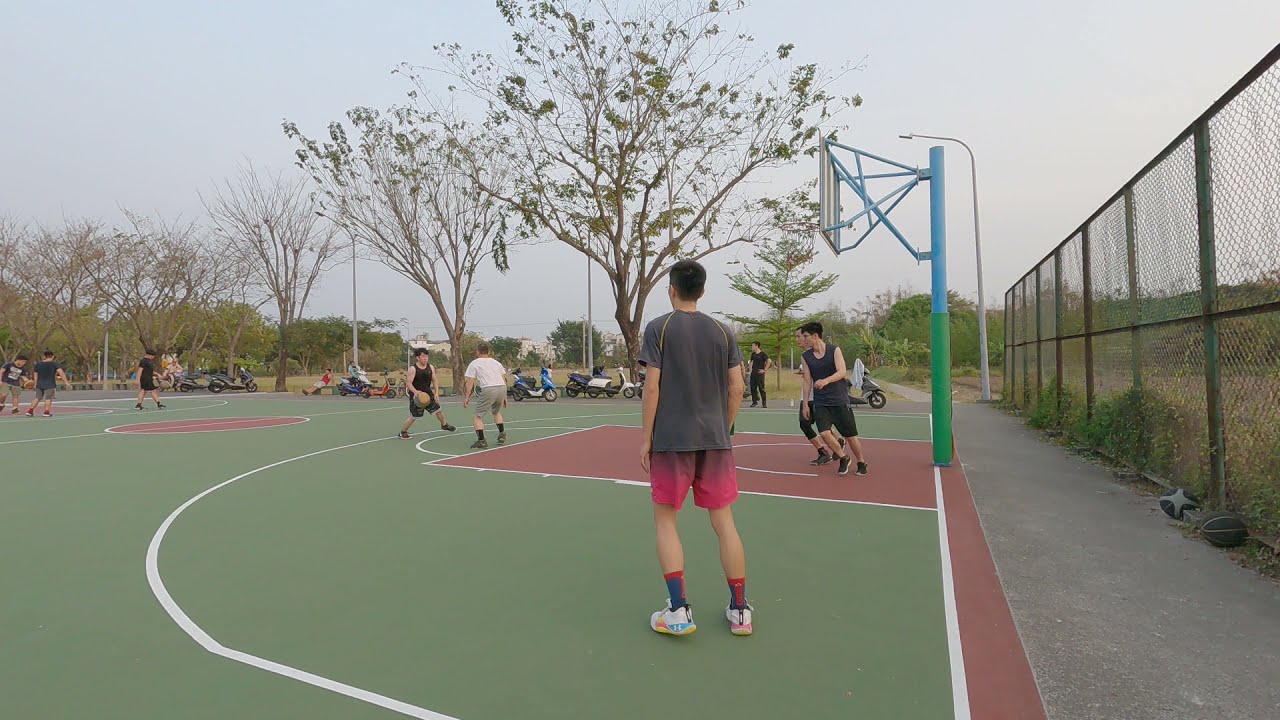In this wide rectangular image, a vibrant scene unfolds at a corner view of a bustling basketball court. The perspective is from the left of the horizontal hoop, which is prominently positioned on the right side of the photograph. The court is vividly colored with green asphalt and areas filled in with red paint, accentuated by white lines marking the play zones. The hoop itself is mounted on a green and blue pole, contrasting against the backdrop.

Five young players, likely older teenagers, engage in an intense game. Two boys position themselves directly beneath the hoop, while two others stand strategically at the free throw line. Another boy, with his back to the camera, is at the forefront of the action. The players are dressed in typical basketball attire: tennis shoes, high socks, shorts, and t-shirts, signifying a casual yet competitive game among friends.

The basketball court is bordered by a tall black gate, beyond which lies a park with slightly dying green grass. The horizon is lined with very tall trees, sparsely adorned with green leaves, hinting at the season being either early spring or fall. A high light post suggests that the court might see activity even at night. Despite occasional mention of motorcycles or mopeds and other possible activities, the scene resonates as a secluded, lively spot where youths gather for the love of basketball, surrounded by nature.